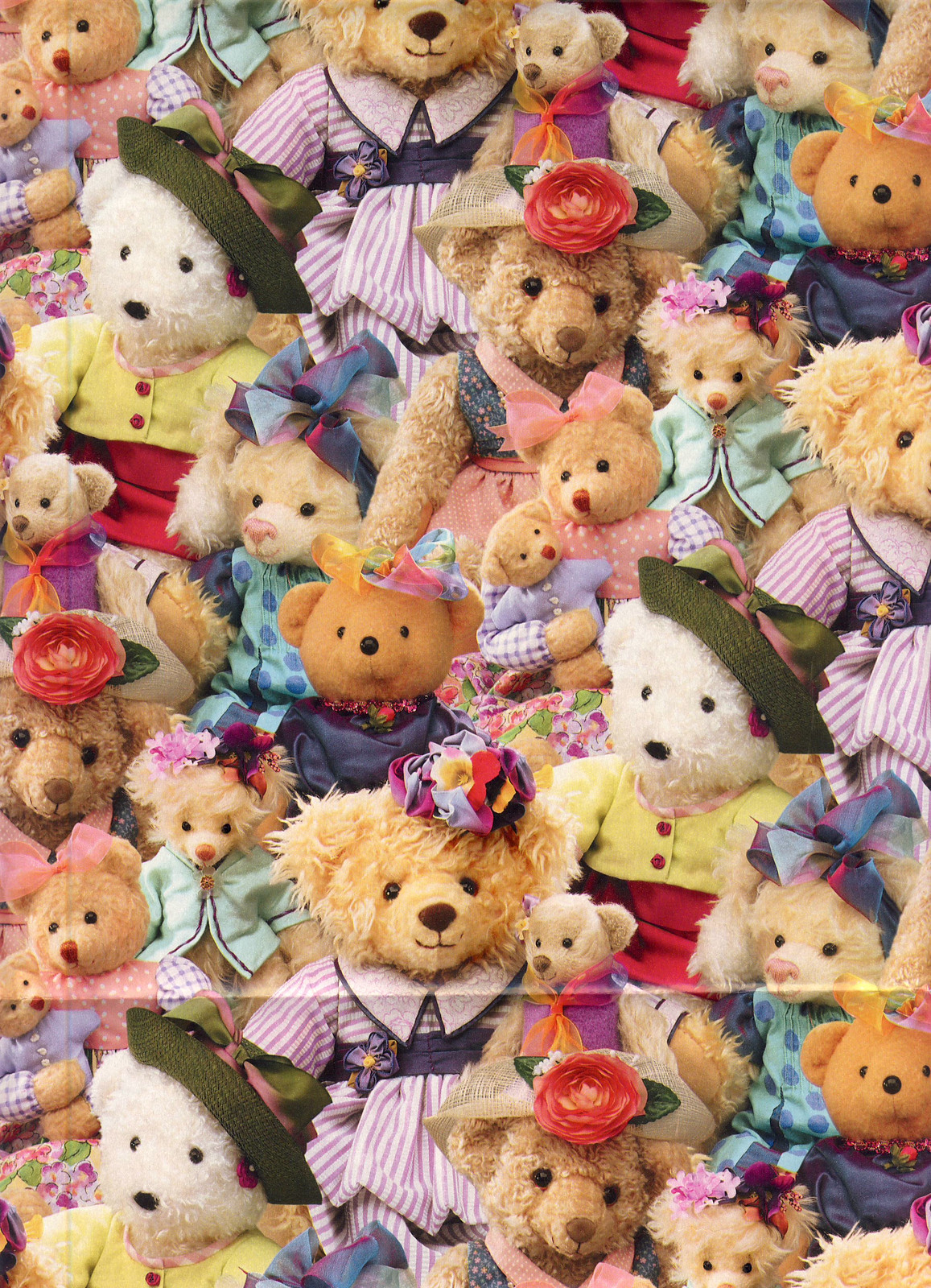The image is a detailed poster featuring a large collection of teddy bears, tightly packed together, filling the entire frame from top to bottom. The teddy bears vary in size, with different fur textures ranging from fluffy to smooth. They come in various colors including blonde, tan, white, and dark brown. Many of the teddy bears are adorned in diverse types of headwear such as party hats, wide brim hats, flowers, and pink bows, and are dressed in human-like clothing including little jackets, dresses, and shirts.

The scene includes several prominent teddy bears: towards the upper section, a mama bear holds a baby bear; nearby, another bear in a pinkish dress also cradles a smaller bear. In the top right corner, a bear with big floppy ears and a white face dons a blue outfit. Below this bear, on the right, there is a bear resembling Winnie the Pooh, donning a dark blue shirt, a small pinkish hat, with black eyes and a black nose. To its left is a smaller fuzzy bear in a green shirt with flowers in its hair. Next to this bear is a larger one in a blue shirt and pink dress, featuring a white hat with a big rose at the center. Further to the left appears a white bear with a tilted green hat, a yellow shirt, and a red skirt.

Some teddy bears appear multiple times throughout the poster, giving a slightly layered impression. Each bear is uniquely characterized, with some identical ones repeating across the poster, adding depth and intricacy to the overall display.